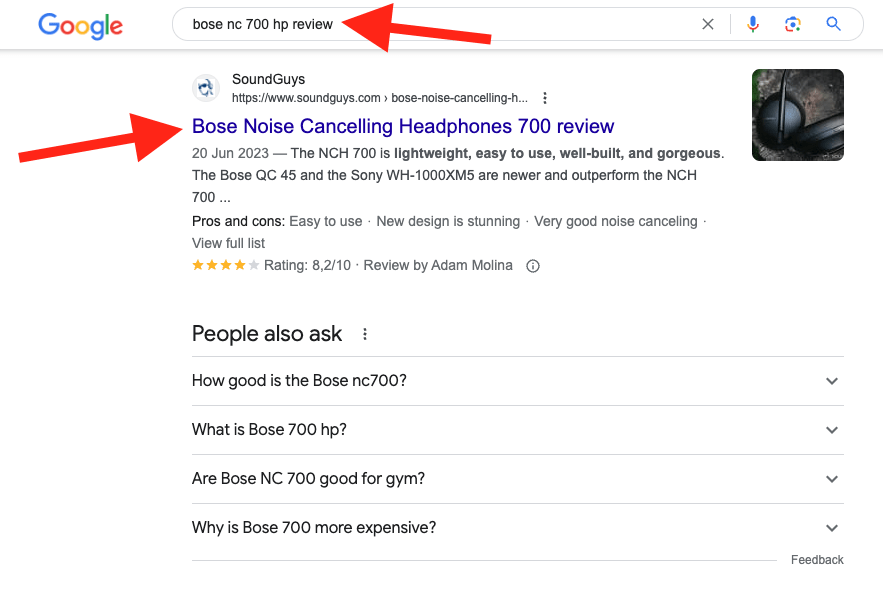The image depicts a Google search results page. At the top left corner, the iconic Google logo is displayed in its signature colors: blue, red, yellow, and green. To the right of the logo, there is a search bar containing the query "Bose NC700HP Review," highlighted by a conspicuous giant red arrow pointing at it. 

On the right side of the search bar, various icons are visible: a small "X" for clearing the search, a microphone for voice search, a refresh button, and a magnifying glass icon denoting search functionality.

Below the search bar, the first search result is from SoundGuys, with the URL www.soundguys.com. In blue text, the title "Bose Noise Canceling Headphones 700 Review" is presented, accompanied by another large red arrow pointing towards it. Directly underneath the title, the date "20 June 2023" is displayed. 

The accompanying snippet details that the NCH700 headphones are "lightweight, easy to use, well built, and gorgeous." It also notes that newer models like the Bose QC45 and the Sony WH-1000XM5 have outperformed the NCH700.

To the right of the text snippet, there is a square image of the black-colored Bose Noise Canceling Headphones 700.